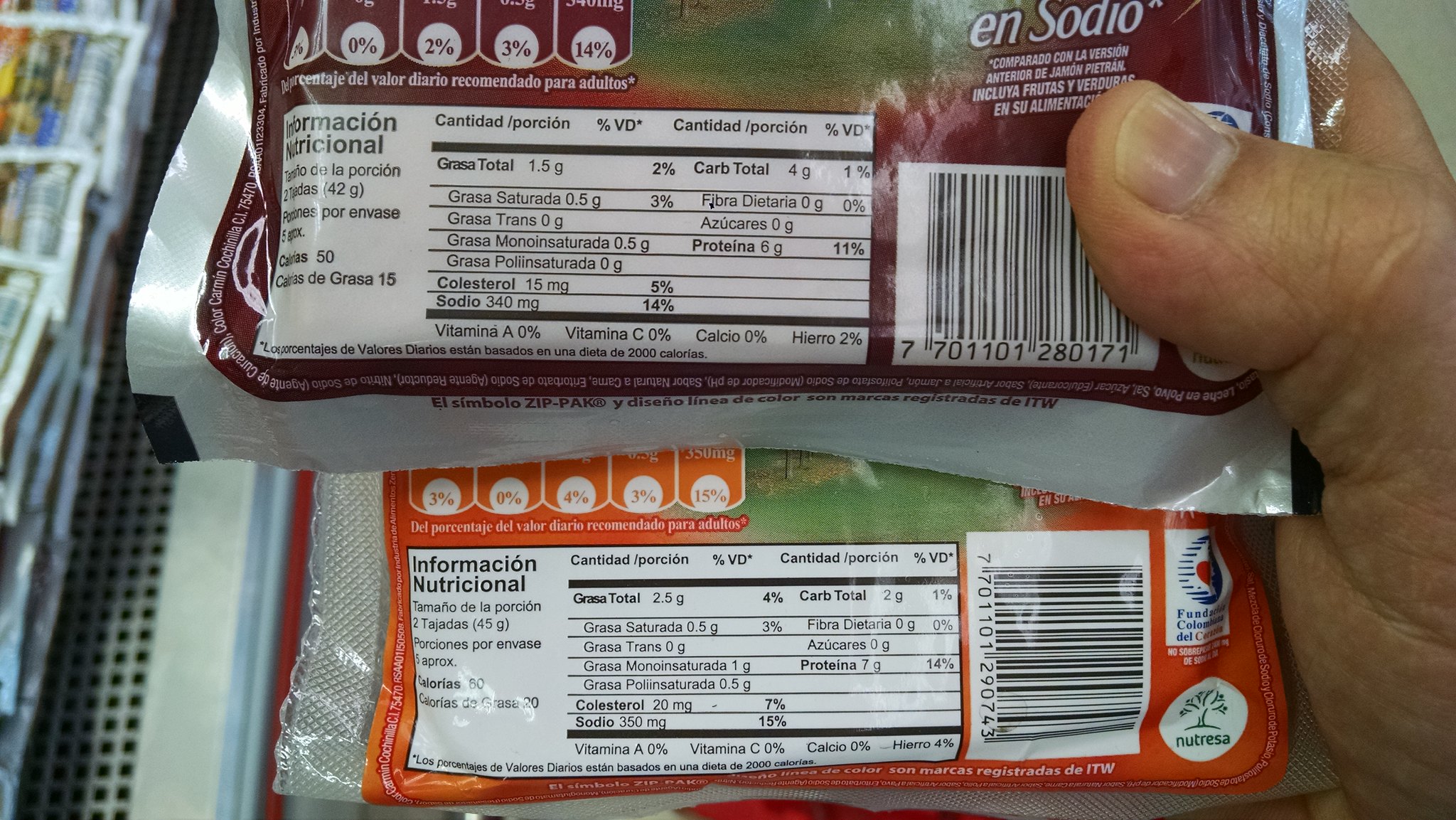This image features the back view of two frozen products, each representing different flavors. Both products are being held up by a man's hand, which is noticeable for its large thumb and a visible scar on the thumb knuckle. The products are likely retrieved from a freezer, as suggested by the presence of a supermarket freezer in the background. The freezer, identifiable by its open, flat design, contains various packaged items, possibly hot dogs, neatly stacked in the upper left section. Although the exact nature of the products isn't discernible from this angle, their packaging features distinct color schemes—green and red for the top product, and green and orange for the bottom one—indicating different flavors and options. The nutritional information is prominently displayed on the back of these products, highlighting their contents and appealing to health-conscious consumers.